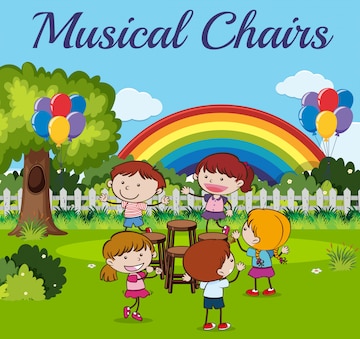The image is a cheerful and vibrant cartoon-style illustration titled "Musical Chairs," depicted in bluish-purple ink at the top. Five children, possibly four girls and one boy, stand around four chairs on a bright green lawn, suggesting they are playing musical chairs. The children, dressed in shorts, skirts, and t-shirts, with a mix of brown and blond hair, and wearing reddish and pinkish shoes, are surrounded by a colorful backdrop. A large, unrealistic rainbow stretches across the light blue sky with fluffy clouds at its base. Multicolored balloons—red, yellow, blue, and purple—flank both sides of the children. To the left, a tree with a hollow, possibly a home for squirrels, adds to the playful scenery, along with a fence and a few bushes, enhancing the illustration's whimsical nature.